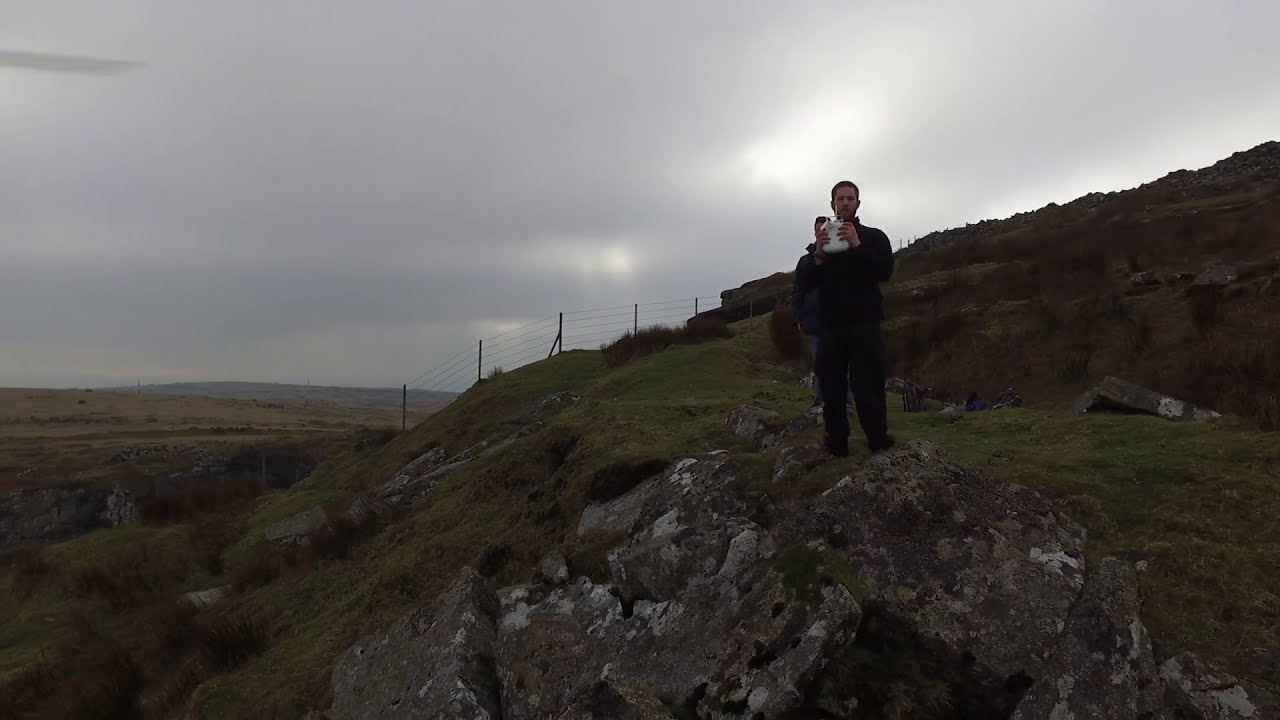The image depicts an outdoor scene on a cloudy, overcast day with a dark, gray sky. Dominating the foreground, a man with light skin stands on a large, gray rock amidst a rocky hillside covered with short grass, low shrubs, and patches of greenery. He is dressed entirely in a dark black long-sleeved top and pants. The man holds up a white remote control device close to his chest, appearing to actively use it. Slightly obscured behind him is another man, partially hidden from view. The hillside overlooks a vast expanse of plains stretching into the distance, with faint, distant mountains visible under the blanket of clouds. Despite a few rays of sunlight struggling to penetrate the thick cloud cover, the overall lighting remains dim and the image somewhat dark.